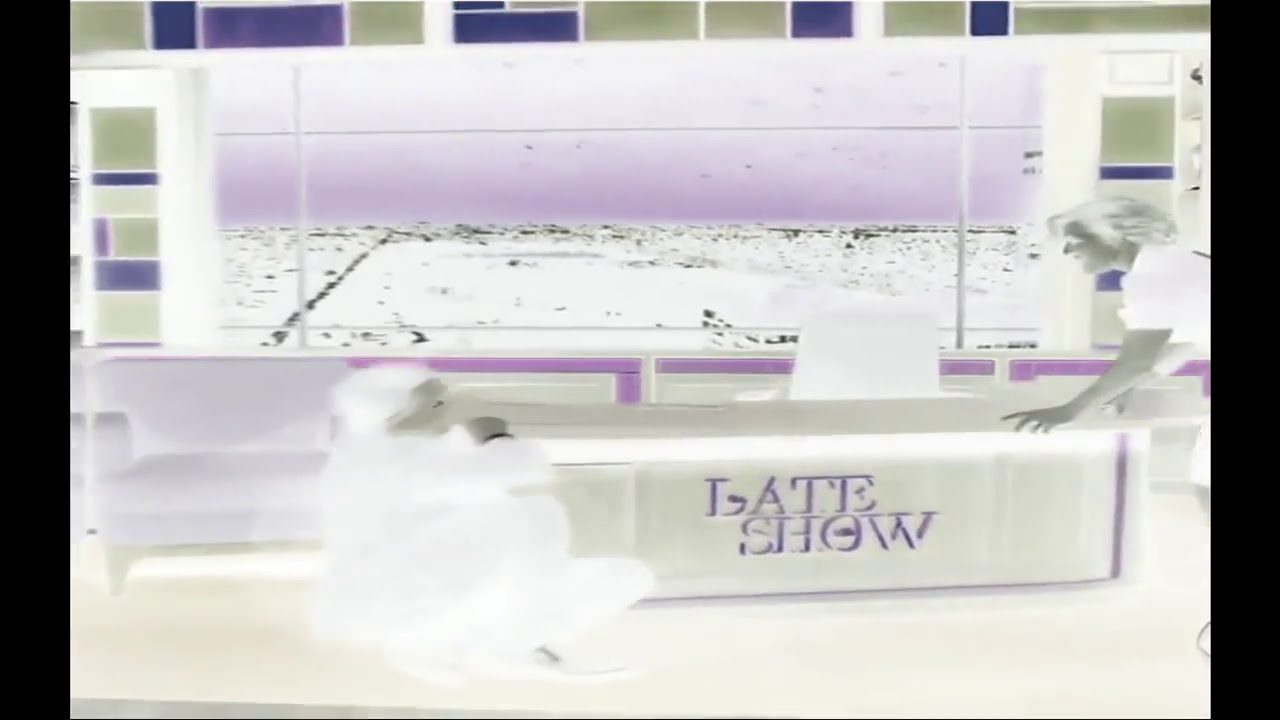The photograph is a horizontally rectangular reverse x-ray type image dominated by grays, purples, and whites. It features a stage set reminiscent of a TV late show, with 'Late Show' text in a serif font prominently displayed on a large desk at the center. The text appears in purple due to the image’s inverted colors. Flanked by black bars on the left and right sides, the scene showcases a detailed, streaky impressionist style. 

On the right side of the image, a woman with white hair and a short-sleeved collared shirt is leaning over the desk, seemingly reaching out. Her skin appears gray due to the inversion effect. Positioned on the floor in front of the desk, a man is either crouching or sitting, looking up at her. Behind them is a backdrop resembling a cityscape, consisting of variously shaded gray and purple rectangles that create an abstract, patchwork-like window scene.

Other elements include a lavender-colored couch on the left side and a puffy chair adjacent to the desk, both add to the impression of a casual yet enigmatic set. The top of the image appears white, which contrasts against the scene's overall dark tones, adding to the ethereal, inverted aesthetic.